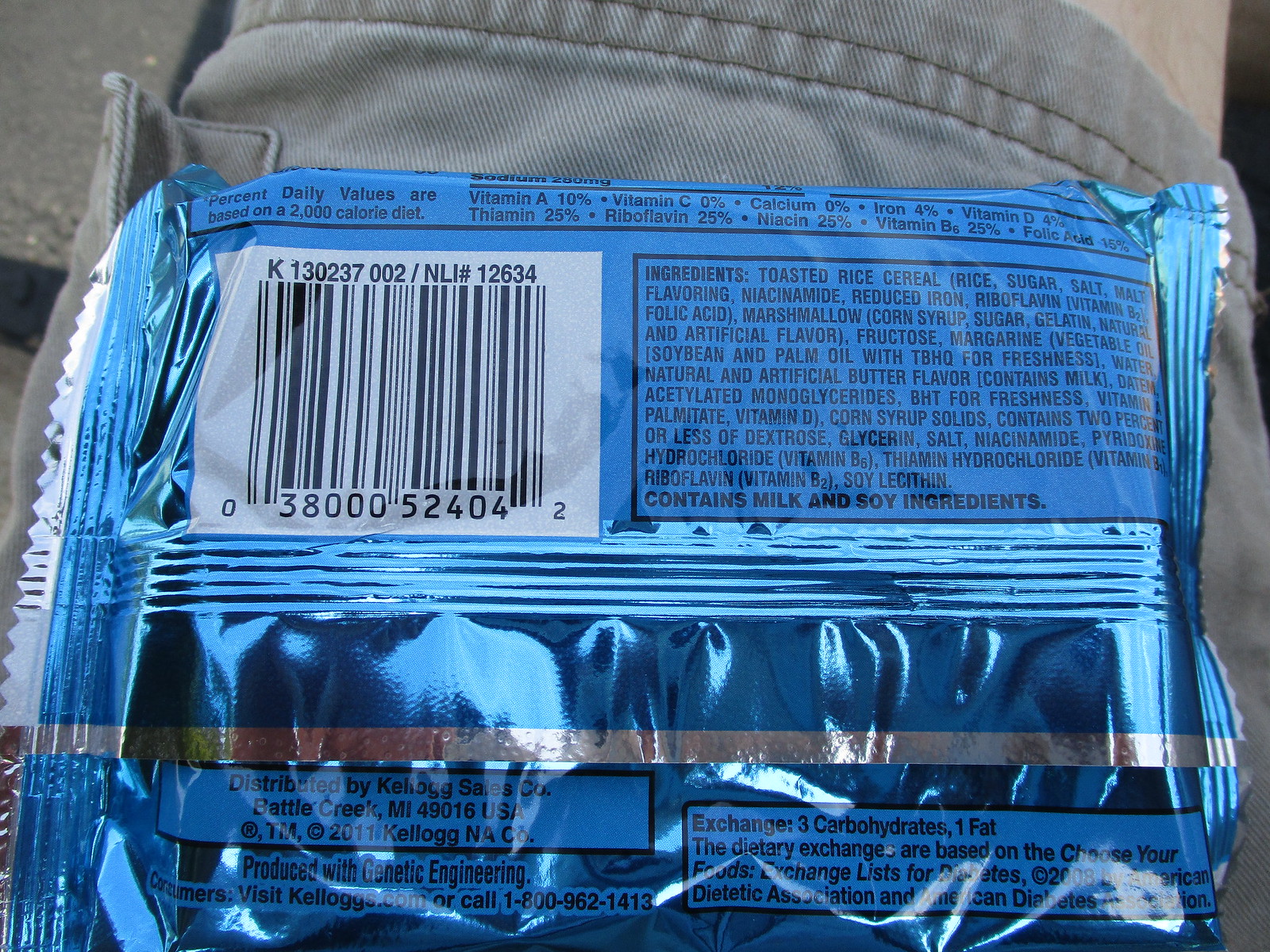In this image, a blue metallic snack bar package is prominently displayed, positioned against the leg of a man wearing light gray denim shorts with side pockets. The focus is on the back of the packaging, preventing the product name from being visible. The package, made by Kellogg's and produced with genetic engineering, features a large black and white barcode on the left side marked with the code K130237002NLI-12634. Above the barcode is a black-outlined rectangle containing nutritional details such as vitamin D, iron, vitamin B, niacin, riboflavin, and thiamine, along with their respective percentages. Below this, another black rectangle boldly lists the ingredients, accompanied by a warning that the product contains milk and soy ingredients. The middle section of the package shows the fold of the wrapping, and at the bottom, a silver band runs horizontally across. Additional rectangles provide further details like the distributor's information, indicating it is Kellogg's Sales Co., along with an address, website, and phone number. The sides of the package feature a silver color, contrasting with the shiny blue of the main body. The detailed layout of the packaging and the legwear provides a comprehensive view of both the snack bar's informational content and the setting of the image.